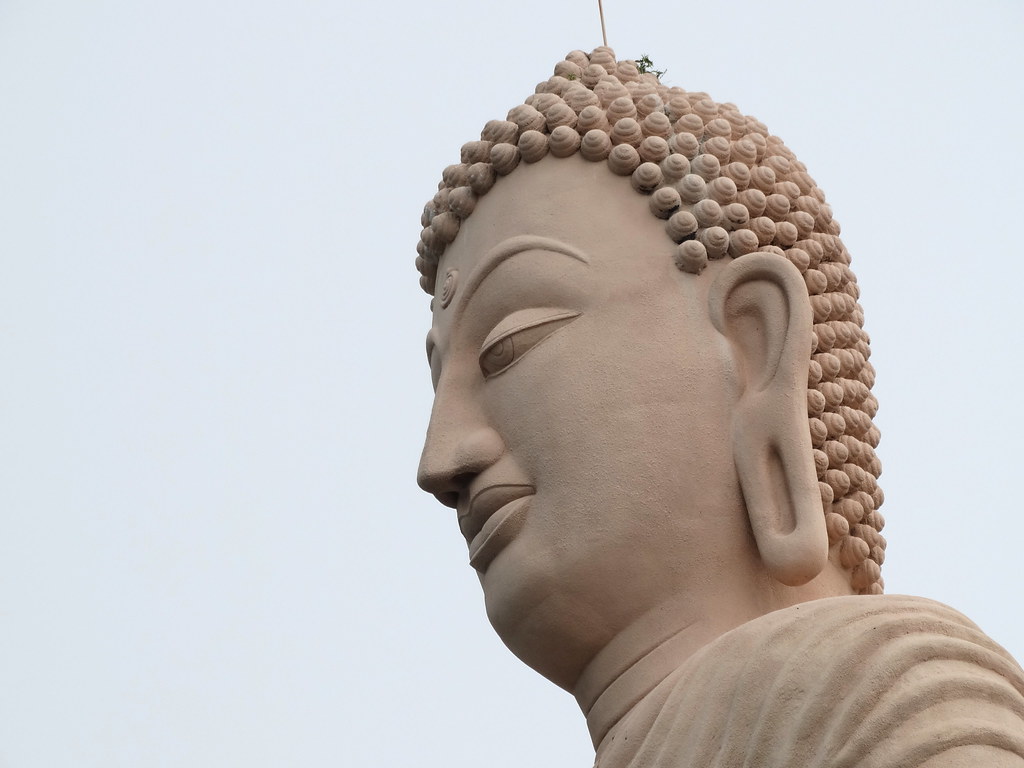The image depicts the head and shoulders of a colossal Buddha statue, standing against a light blue or gray sky, suggesting an overcast day or the approach of dusk. The statue is a light tan or beige color, with subtle differences only in the hair, which is darker. The hair is intricately crafted into tiny curls or half seashell-like shapes that cover the head from the forehead to the neck. A circular jewel adorns the center of the forehead. The Buddha's eyes appear half-closed, giving a serene expression, while the nose is prominently projected and the lips are large and pursed. The earlobes are notably elongated with drooping oval-shaped gauge holes. Draped over the Buddha's left shoulder is a folded robe, intricately detailed and part of the same material as the statue itself, emphasizing the craftsmanship. This striking statue, viewed from below, emphasizes its grandeur against the soft hue of the sky, reinforcing its imposing presence.